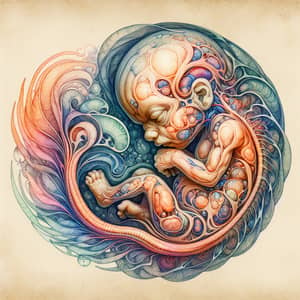This is a highly detailed drawing or painting that vividly depicts a nearly fully-grown human fetus in utero. The fetus, with its prominent head and developed features, is positioned in the classic fetal pose with eyes closed, elbows bent, and one hand resting against its face, while its knee is drawn up towards its left hand, giving a clear left-side profile view. Through the translucent depiction of its body, intricate details such as outlined muscles and visible brain can be seen. The fetus is encased in a vibrant, rainbow-colored amniotic sac featuring hues of orange, red, purple, yellow, green, and blue. The composition is set against a light brown, square background that adds a contrasting simplicity to the complex, colorful elements within the womb. The artistry showcases a blend of naturalistic and somewhat surreal elements, emphasizing both the wonder and complexity of the beginning stages of human life. The overall impression is one of celebration and intricate beauty, with the medium appearing to be a fusion of traditional drawing techniques and digital artwork. There is no text present in the artwork.